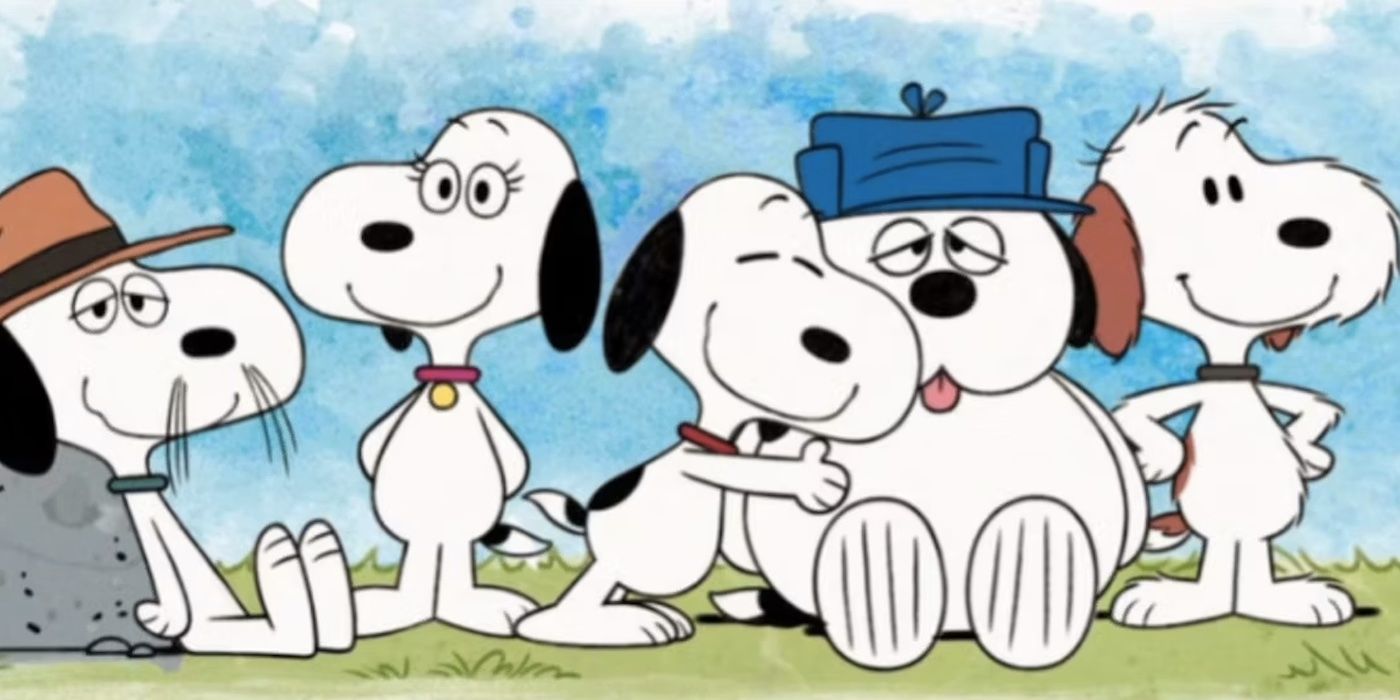The image is a colorful animated cartoon featuring various renditions of Snoopy set against a backdrop of a blue sky. From left to right, there are five Snoopy-like characters. The first Snoopy is leaning against a rock wearing a brown hat and has whiskers protruding from his nose. Next is a Snoopy with long eyelashes, a red collar with a gold tag, standing and smiling. The central figure depicts Snoopy with closed eyes and a huge smile, joyfully hugging a larger, chubbier dog who is sitting down. This larger dog sports a blue hat, has cross-eyed or sleepy-looking eyes, and his tongue hanging out. To his right, there is another fuzzy Snoopy with brown ears and spots, hands on his hips, smiling. Each Snoopy variant reflects different characteristics while maintaining the iconic charm of the original character.